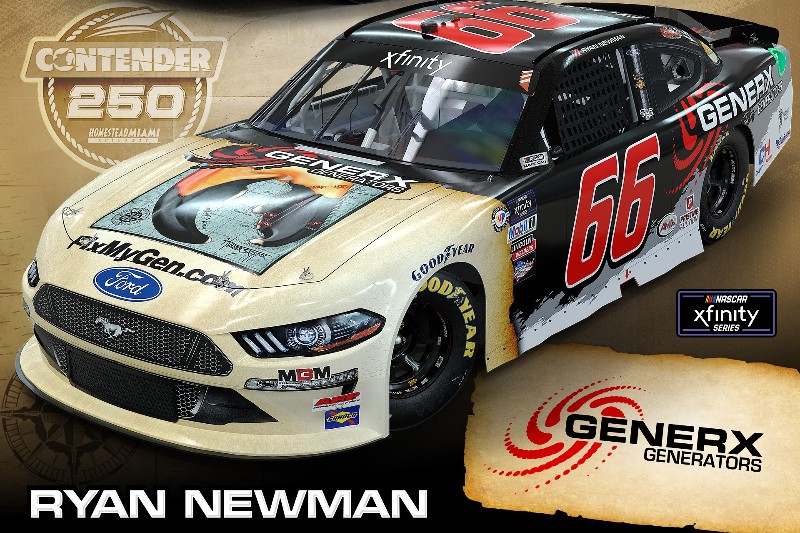This vividly detailed digital poster features a striking image of a high-performance Ford Mustang race car, emblazoned with the number 66 in bold red on its doors and roof. The car's dynamic design showcases a sleek white front transitioning to a black rear, adorned with numerous sponsor logos from companies like MGM, FixMyGen.com, and Ford. Prominent Goodyear branding decorates the tires in yellow, reinforcing its status as a race-ready vehicle.

Centrally positioned on the car is the iconic Ford Mustang horse logo, reinforcing its sporty lineage. The backdrop of the image is a contrasting brown ground which sets off the car's sleek lines. In the top left corner, a circular logo reads "Contender 250," hinting at the car's participation in a competitive racing event. The lower right corner of the poster prominently displays the "Xfinity Series NASCAR" logo above the "GenerX Generators" logo, showcasing additional key sponsors.

At the bottom left, the driver’s name, Ryan Newman, is inscribed in white, cementing his association with this high-powered machine. This advertisement expertly combines all key elements of sponsorship and racing prestige to capture the viewer's attention.